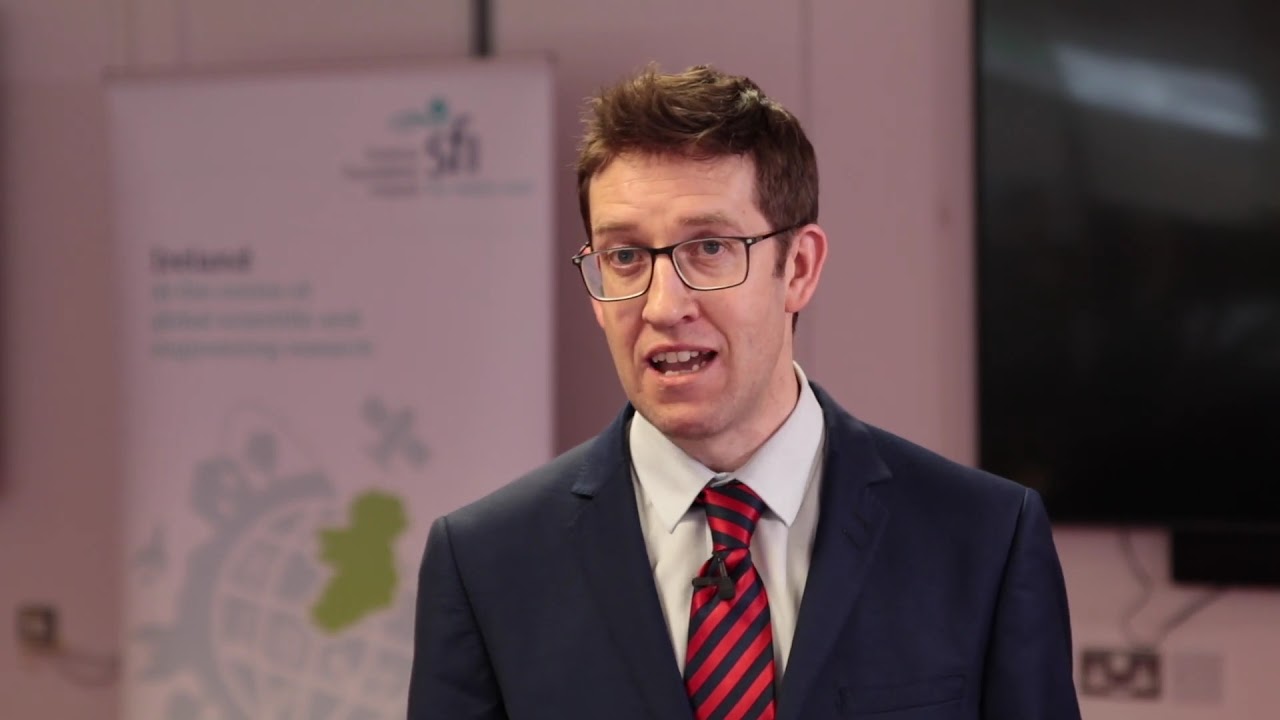The photograph captures a middle-aged white man with slightly messy, short brown hair styled upwards at the front. He is wearing rectangular black-rimmed glasses and a white dress shirt underneath a navy suit coat. His red and navy blue diagonally striped tie features a small clip microphone. The man is positioned in the sharp, focused foreground, mid-speech with his teeth visible. The background is slightly blurred, featuring a suspended informational banner with a graphical design of a globe and some unreadable text, giving an impression of a corporate event or training. To the right, a large, unlit flat-screen TV is mounted on the wall with a cord protruding from the bottom.